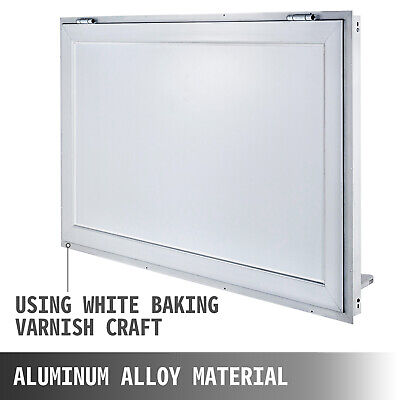This image displays a rectangular, white object prominently against a pure white background. The object appears to be a cabinet or cover with a door that opens upwards, secured by two silver hinges at the top. There is a small silver chain hanging from the bottom left corner of the cabinet. Notably, there is no writing on the object itself. However, there are two blocks of text on the image: one above stating "using white baking varnish craft," and another below indicating "aluminum alloy material." At the back right corner near the bottom of the object, a smaller white rectangle protrudes. The bottom foreground of the image features a gradient rectangle transitioning from black on the left to white on the right, with the words "aluminum alloy material" displayed in large, white blocky text. The minimalistic design of the photograph and description suggests it may be a part of an advertisement for the product, though specific uses are not detailed.